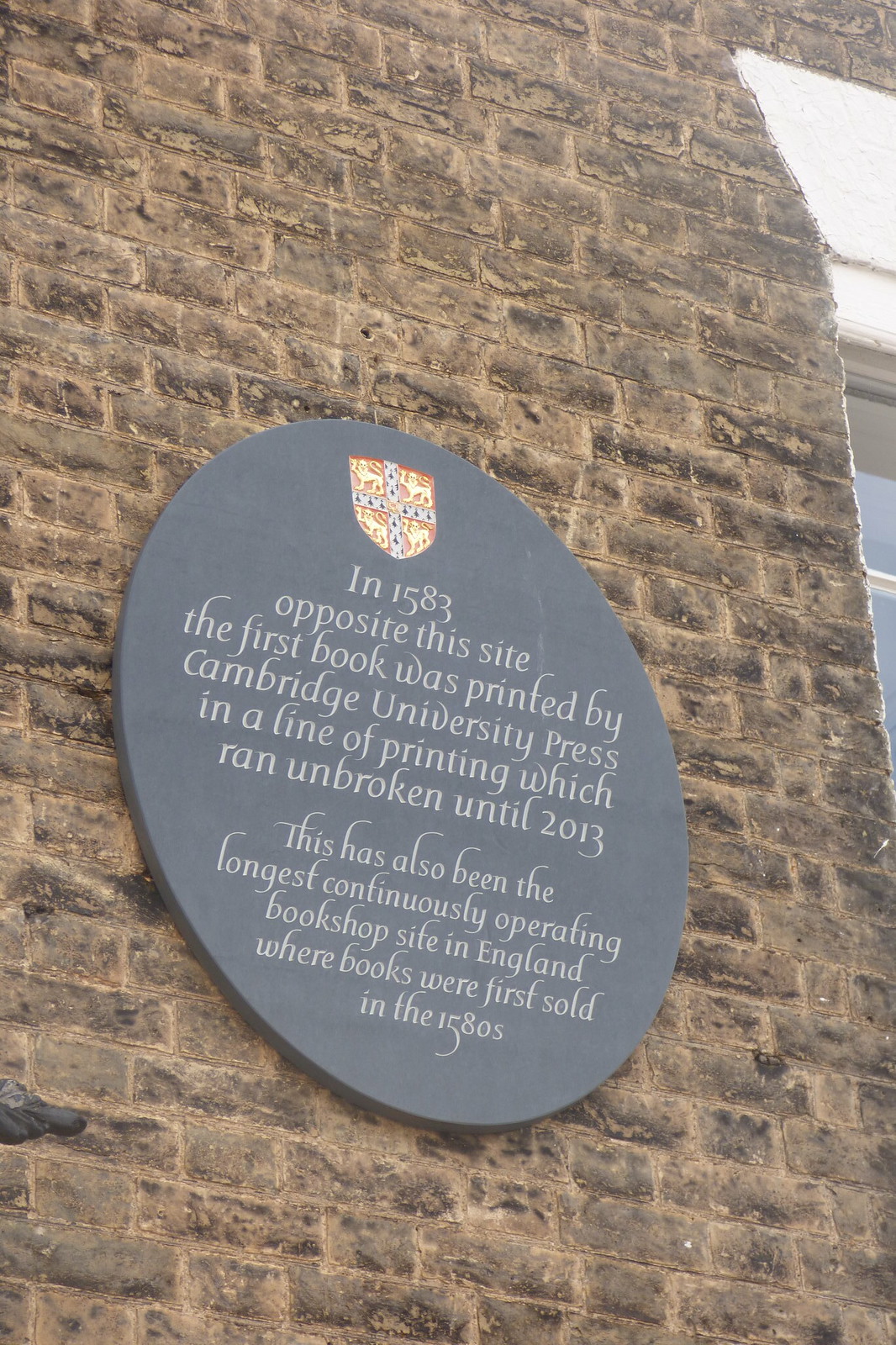This photograph depicts a circular modern gray sign affixed to the weathered, beige, and worn stone wall of an old building. At the top of the sign is a coat of arms in yellow, red, and gray. Below the coat of arms, the sign reads, "In 1583, opposite this site, the first book was printed by Cambridge University Press in a line of printing which ran unbroken until 2013." The sign further states in a slightly smaller, ornate script that, "This has also been the longest continuously operating bookshop site in England, where books were first sold in the 1580s." The worn stones and the historical context provided by the sign highlight the significant heritage of the site.